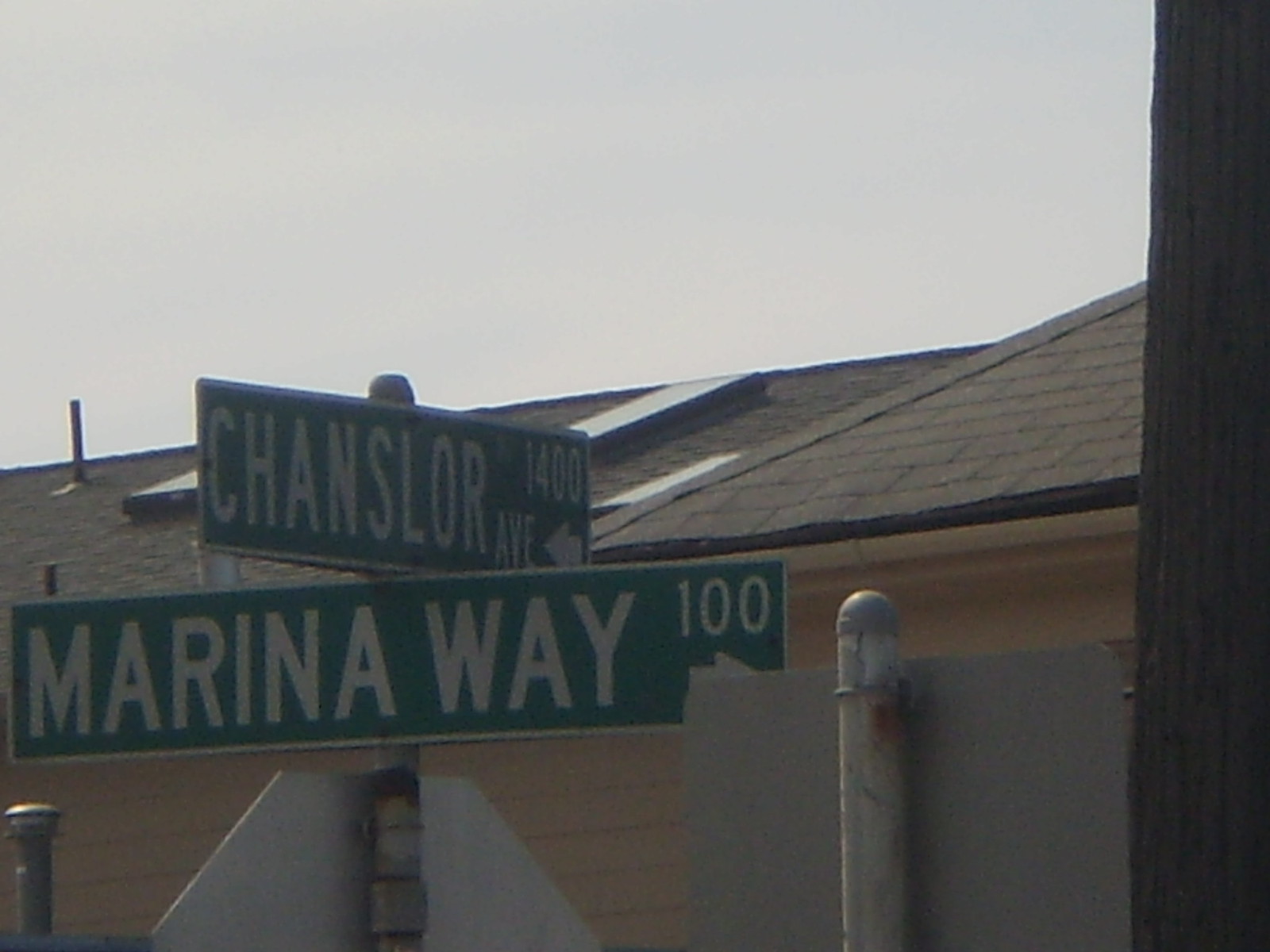This daytime photograph captures a detailed urban scene featuring various street signs and elements of the surrounding architecture. In the foreground, the white back of a stop sign is prominently displayed. Above it, two green and white directional signs are mounted: the lower sign reads "Marina Way 100" with an arrow indicating direction, while the upper sign reads "Chancellor Avenue 1400" with its own directional arrow. The background reveals the grainy texture of a light gray sky and a granny-colored siding on a nearby building with a brown roof accented by a visible silver smokestack. The picture also shows the back of another metallic sign and the wood grain of what appears to be either a power pole or a tree. Both signs exhibit notable reddish-brown rust spots. The photograph has a slight graininess, adding a touch of texture to the image.